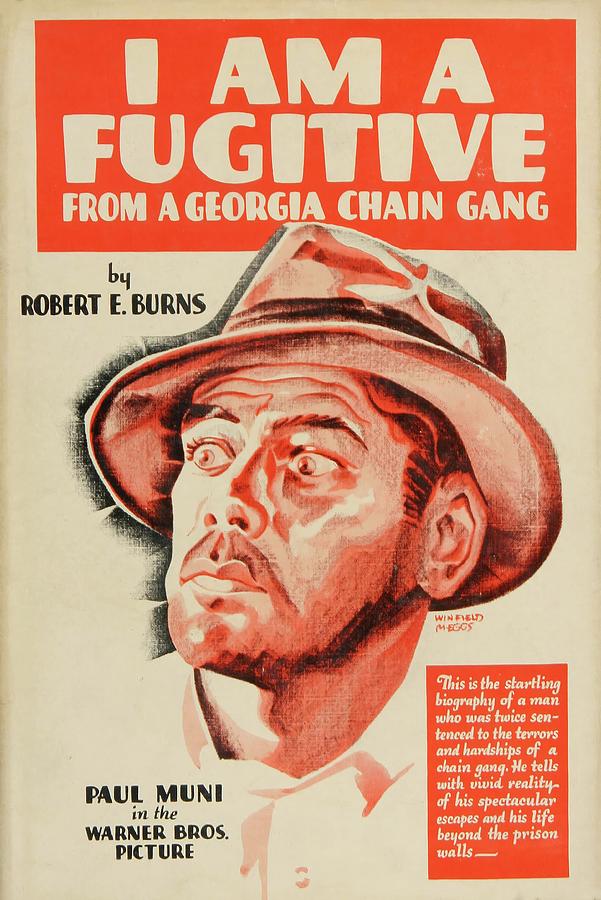The image is an advertisement for a classic movie titled "I Am a Fugitive from a Georgia Chain Gang." The background is predominantly orange, with the title written at the top in beige text. Below the title, in black text, it reads "by Robert E. Burns." Positioned to the right midsection is a prominently drawn portrait of a man, who appears surprised, with wide-open eyes. He is wearing a fedora, colored in an orangish-white hue with a black stripe around the top. The man is angled to the right, with light reflecting off his visage, emphasizing his expressions. Below the illustration, it reads "Paul Mooney in the Warner Brothers Picture" in black text. On the right-hand side, a paragraph in small, white cursive text describes the content: "This is the startling biography of a man who was twice sentenced to the terrors and hardships of a chain gang. He tells with vivid reality of his spectacular escapes and his life beyond the prison walls." The overall design features a lot of bright, orange color, making it visually striking.